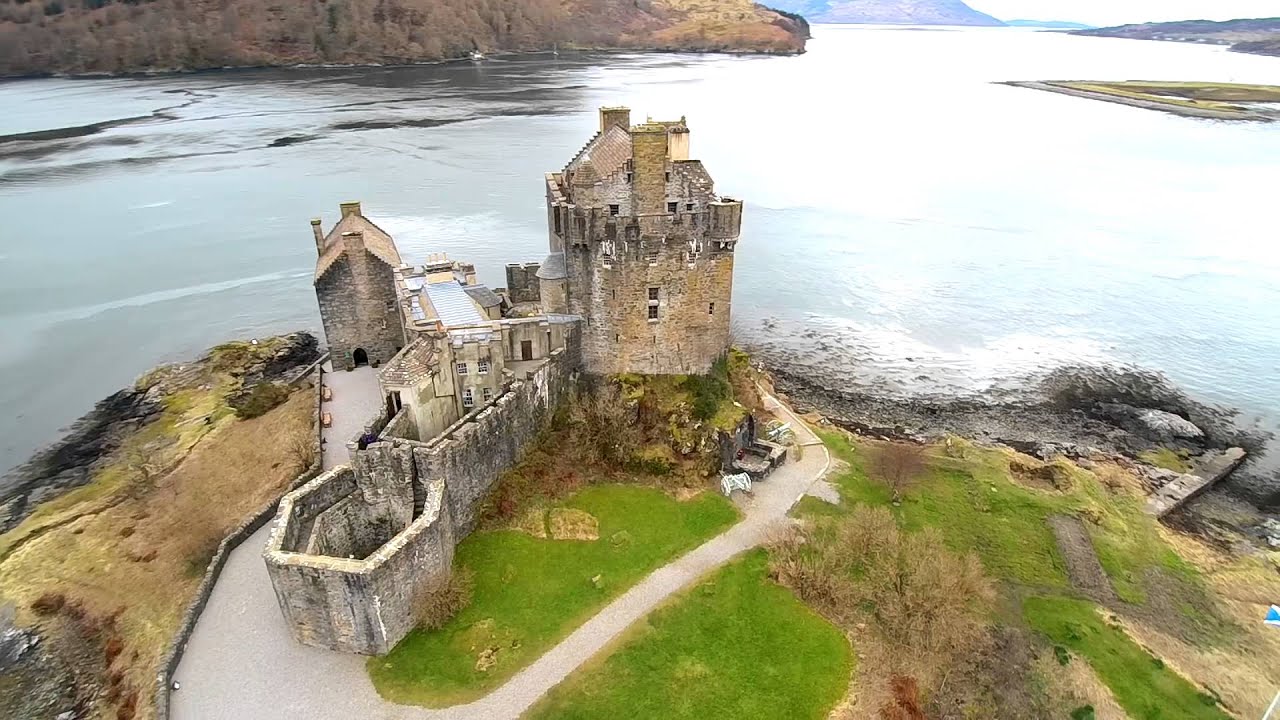This landscape photograph, likely taken in the United Kingdom, captures an aerial view of a majestic and rugged castle perched on a small outcropping of land at the edge of a large body of water, possibly the ocean. The castle, constructed from dark tan stone, stands tall with its battlements prominently tracing the top. It is a complex structure with multiple attached buildings, including a prominent stone house atop the main edifice. A winding driveway leads up to the castle, which appears to be surrounded by lush, green grass. The castle complex extends to the left and behind, featuring additional stone structures and a smaller house. To the left side of the photograph, beyond the castle, a steep rock cliff juts out, with more distant hills and blue-tinged mountains visible in the background. The rugged coastline contrasts vividly with the smooth expanse of water, where waves are seen hitting the rocks at the shoreline, conveying a serene yet formidable scene.